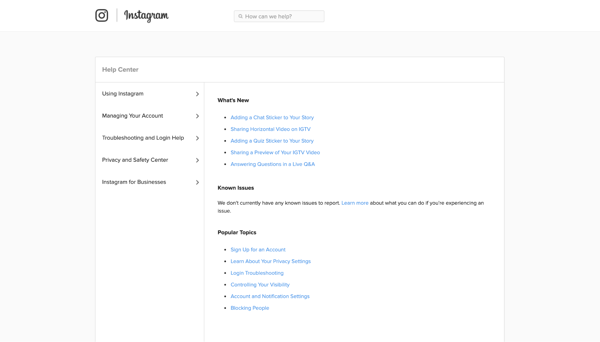This screenshot captures the Instagram Help Center as viewed on a desktop device, likely a computer or laptop, indicated by the wide screen format and the Instagram logo positioned distinctly in the top left corner. The interface presents a structured layout typical of desktop browsing. The user has specifically navigated to the Help Center section on Instagram's website. 

Prominently displayed, the Help Center features a main heading titled "What's New" followed by five subheadings in blue, each serving as hyperlinks to different parts of Instagram for detailed assistance. Below these, a subtitle, "Popular Topics," organizes additional information into six more hyperlinked subheadings, also styled in the same blue font. 

On the sidebar to the left, the navigation options include "Manage Your Account," "Troubleshoot and Login Help," and "Instagram for Businesses," offering users specialized pathways to address their specific needs. This detailed layout suggests a well-organized support system accessible directly from the desktop environment.